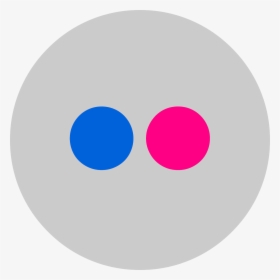The image features a perfectly square, light-gray background. Centrally positioned within this square is a slightly darker gray circle. This circle is small enough that it nearly touches, but does not quite reach, the edges of the square. Inside this gray circle, there are two smaller, colored circles: a blue one on the left and a red one on the right. Both of these smaller circles are precisely aligned on the horizontal centerline of the gray square, maintaining perfect horizontal symmetry. The blue circle is placed just to the left of the vertical midline, whereas the red circle is just to the right of it. The composition is clean and minimalistic, featuring only these elements against the monochrome background.